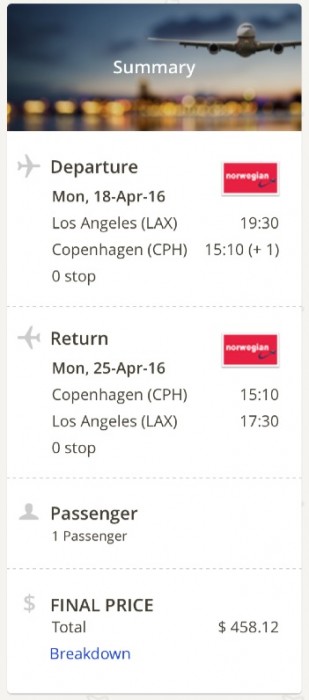The mobile screenshot displays detailed flight information for a round trip between Los Angeles (LAX) and Copenhagen. At the top of the image, there is a picture of an airplane either taking off or landing, set against a predominantly dark blue sky with visible clouds. The airplane is positioned on the right side of the image and is white in color. Overlaid text in the center reads "submarine light."

Following this, the image transitions into a section with a white background. It starts with gray-colored airplane icon pointing to the right. The text accompanying this icon details the departure information: "Departure: Monday, 18 April 16, Los Angeles LAX, 19:30, Copenhagen 15:10 +1, zero stop." On the right side of this information is a red square with the word "Norwegian," indicating the airline.

Below this, another section features a gray airplane icon pointing to the left, indicating the return flight. The text here reads: "Return: Monday, 25 April 16, Copenhagen 15:70, Los Angeles 17:30, zero stop." The same red Norwegian Airline logo appears on the right side.

Further down, an outline of a person next to the word "Passenger" signifies passenger information. Below this, it reads "one passenger." Additionally, there is a gray dollar sign icon followed by the text "Final Price: Total $4.5812." The latter part of the text reflects a commentary on the pricing, noting, “dang, that’s pretty cheap from LAX to Copenhagen, who’d have thought?”

The screenshot provides a comprehensive view of the travel itinerary, fare, and airline details, all succinctly laid out for easy interpretation.